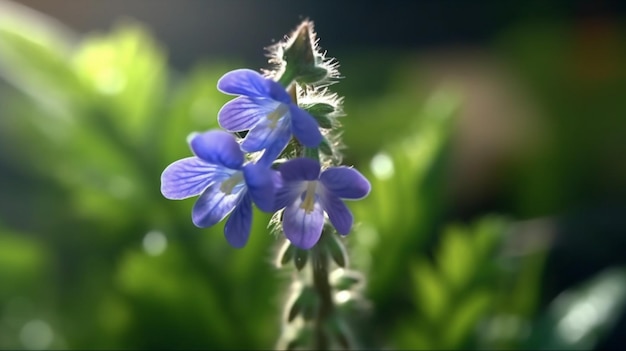This close-up, horizontally oriented photograph captures three light purple flowers atop a green stalk, each adorned with five rounded petals—though a couple have six petals. The petals display a delicate medium-purple hue with deeper purple veins, and their inner portions are white. Each flower features two long, white stamens with yellow tips rising from the center. The green stalk is covered with fine white hairs and flanked by small, oval-shaped leaves. In the blurred background, a sunlit array of green, fern-like and other indistinguishable leaves create a glistening, lush backdrop. A dark area appears in the top right corner, adding depth to the composition.